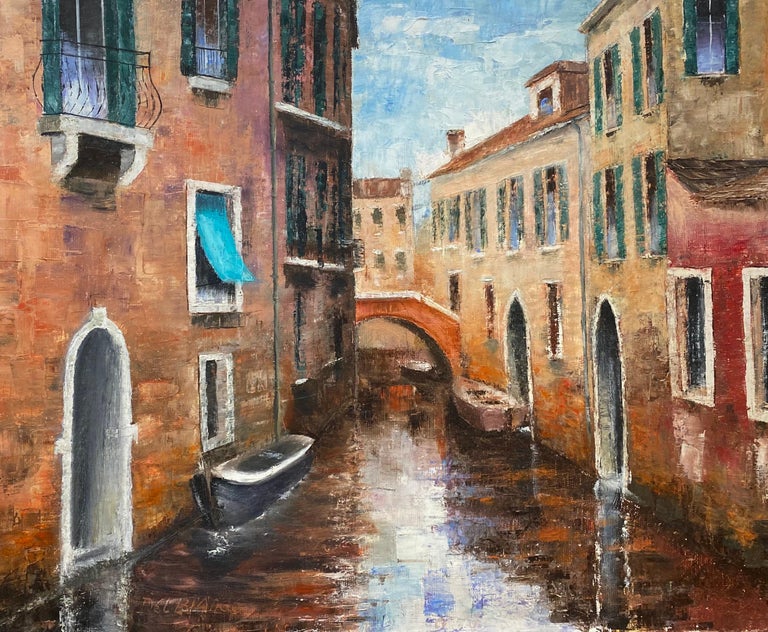This impressionist painting of Venice captures a serene waterway flanked by two picturesque buildings. On the left, a three-story brown structure showcases an arch-shaped white entrance towards the left, with a second-floor window adorned with blue curtains and a small black metal balcony. In front of this building, a black bulge is visible. The building on the right features a blend of brown and red hues, complemented by two arch-shaped entrances. Both buildings reflect a gradient from a dirty orange near the water to a lighter yellow higher up. Far in the background, a bridge connects these two structures, drawing the eye across the scene. The river itself is depicted in shades of brown, with a striking white, shiny reflection in the middle, adding depth and movement to the tranquil waterway. Small boats are parked outside some doorways, enhancing the Venetian charm.